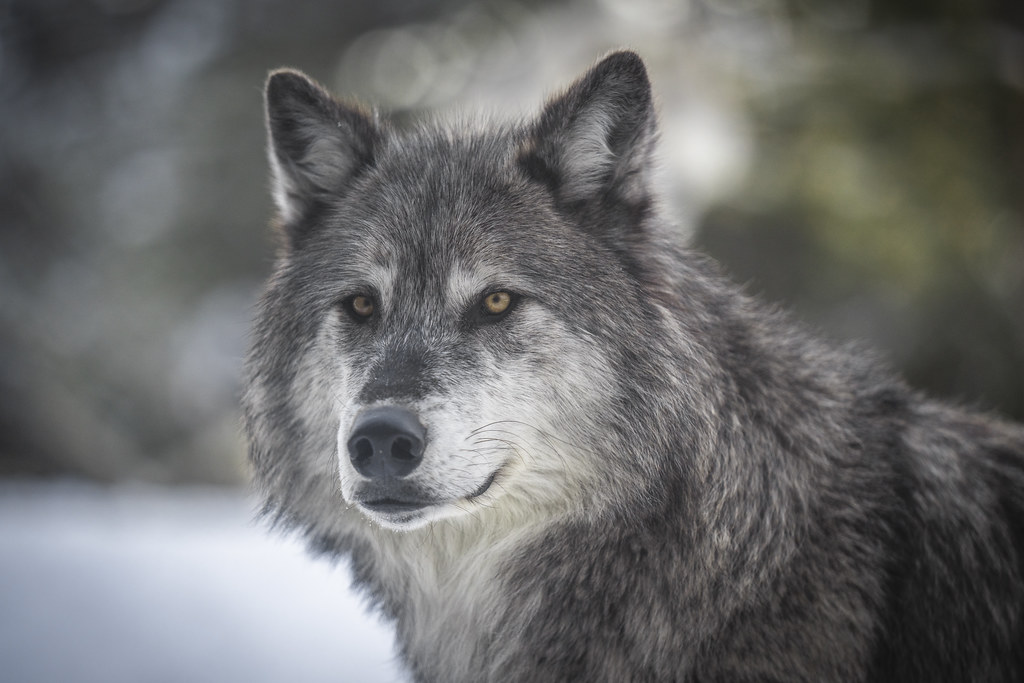This professionally taken artistic photograph features a close-up of a wolf, centrally focused, showcasing a detailed portrayal of its head and upper torso. The wolf's fur is a thick mix of gray, white, and light black, with white markings prominently visible alongside its nose and underneath its belly. Its eyes are a striking amber or light honey golden color, exuding a predatory focus as it gazes slightly to the left of the viewer. The wolf's ears mirror the color pattern of its body with white interiors and black-tipped tops. 

The background is softly blurred, suggesting a snowy environment with potential trees, adding a pastel hue and soft lighting that enhances the texture of the wolf's fur. This element, coupled with the overall composition, lends the photograph a sense of character and beauty, making it seem taken during a tranquil moment in a winter forest.